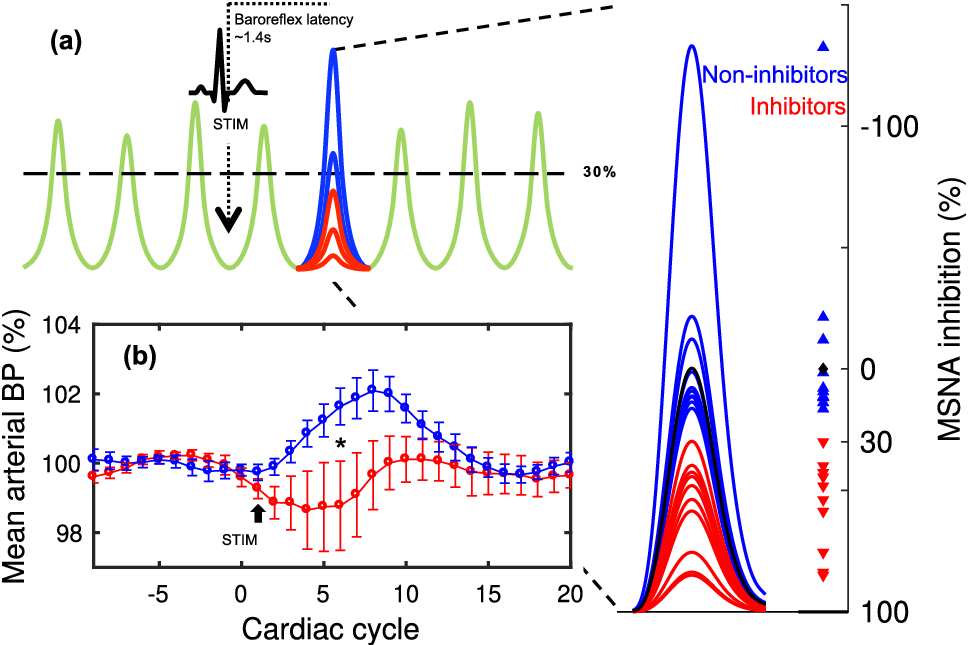This image is a detailed, computer-based medical display, potentially used in medical schools or science classes, depicting three distinct charts related to cardiovascular function. The primary chart, labeled "Baroreflex Latency," features a consistent green sinusoidal wave that spikes up and down, occasionally changing to blue and red in the center section. This wave represents heart rhythms tracked across a "cardiac cycle" on the x-axis and "mean arterial BP (percentage)" on the y-axis.

Below this, there are intersecting red and blue lines labeled clearly within the chart, continuing the cardiovascular analysis by showing variations in mean arterial blood pressure. On the far right, a third chart illustrates different groups indicated by "Non-inhibitors" in blue and "Inhibitors" in red, with blue lines peaking higher than the red and black lines. This chart measures "MSNA inhibition (percentage)," highlighting a comparative analysis where a blue spike surpasses a red spike, emphasizing the differences in inhibition levels across groups.